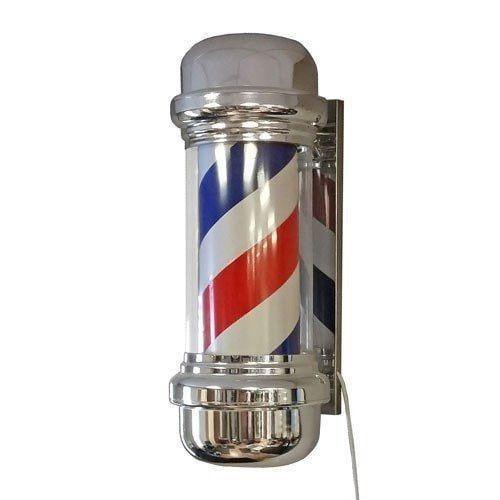In the center of a photo with an empty white background stands a classic barbershop pole, typically found outside barbershops. This pole, a quintessential symbol of barbering, features spiraling stripes of red, white, and blue that run diagonally along its cylindrical, see-through glass body. The pole is mounted on a reflective silver metal bracket attached to a flat plate, which is likely fixed to the wall of a barbershop. Topping and base sections of the pole are marked with silver caps—the top cap appears dull gray. A small wire, possibly for powering the rotation mechanism, is visible at the bottom of the mounting plate. The clean, metallic finish and vibrant colors give the barber pole a shiny, almost new appearance.